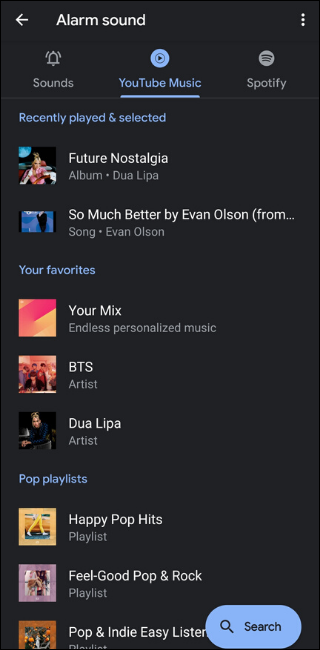The image depicts a dark-themed search interface, presumably on a mobile device set to dark mode. At the top of the screen, there is a search bar where the user has entered the query "alarm sounds." Just below the search bar, three navigation tabs labeled "Sounds," "YouTube Music," and "Spotify" are displayed. The "YouTube Music" tab is highlighted in blue, indicating it is currently selected.

Underneath the navigation tabs are the search results, categorized into different sections. The first section, labeled "Recently Played," displays two songs that the user has recently listened to. Following this, there's a section titled "Your Favorites," showcasing three songs that the user has previously marked as favorites. The next section, "Pop Playlists," features three different playlists within the pop genre.

Each section—whether it's "Recently Played," "Your Favorites," or "Pop Playlists"—contains a mix of album covers, individual songs, artist names, and playlists, visually represented through small thumbnail images. This detailed layout allows the user to quickly navigate through their musical preferences and find specific alarm sounds efficiently.